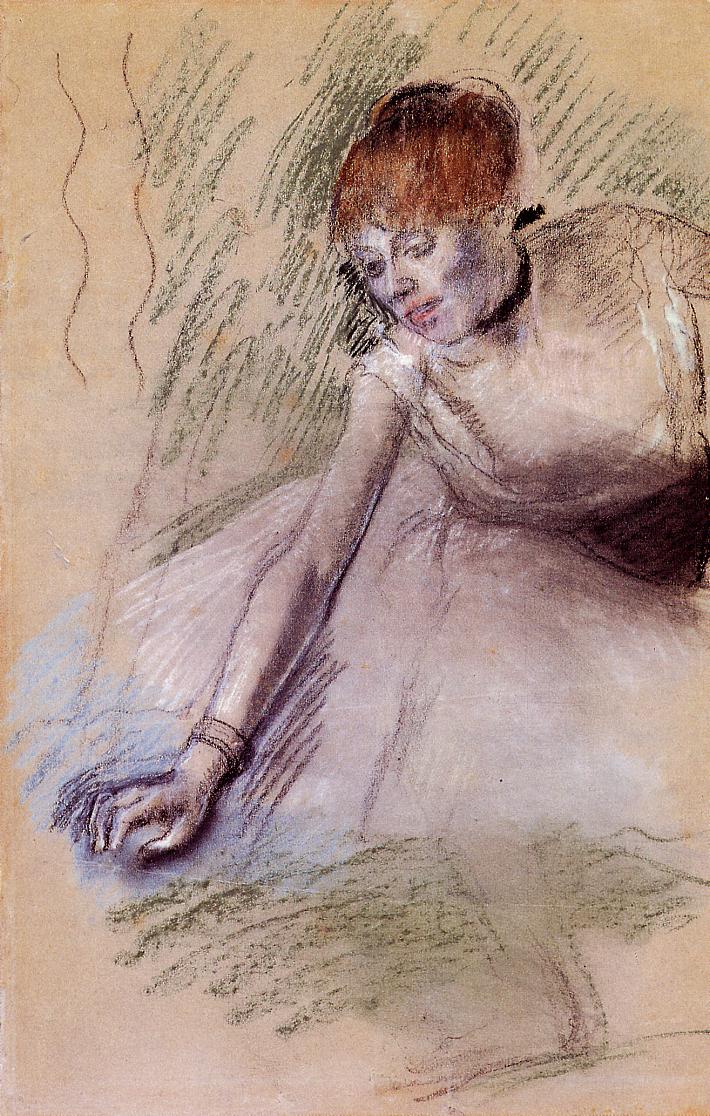This is a detailed sketch of a woman rendered in an abstract style. Her appearance is disheveled, reminiscent of the Princess Bride, with red-brown, bowl-cut hair that does not extend past her ears. Her facial features are the most detailed part of the artwork, showcasing blackened cheeks, downcast eyes, a well-defined nose, and red lips adorned with makeup. She wears a short-sleeved white gown or dress, complemented by a bracelet on her right arm. The pose suggests she is on the verge of collapsing, possibly leaning on her right arm for support, as if she's about to fall or grasp something not clearly depicted in the drawing. The background and areas surrounding her form are filled with sketch marks and green scribbles, further enhancing the abstract nature of the piece.